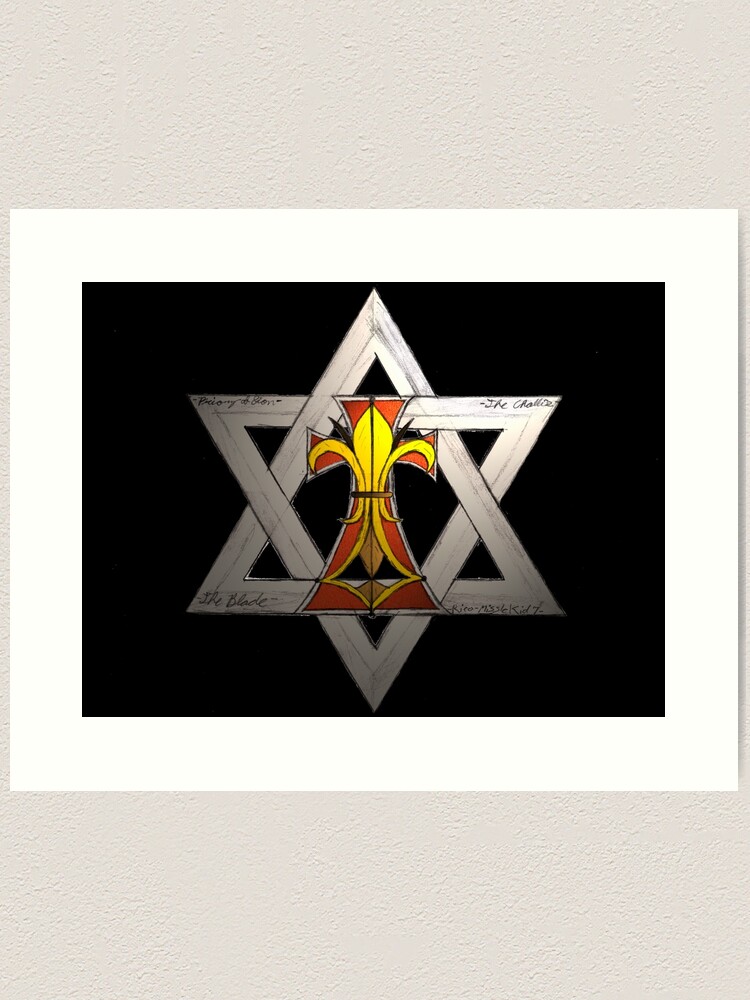The image depicts a digitally created geometric star composed of two interlocking triangles, one pointing up and the other down, against a black background with a white and tan border. The star is white and features a centrally placed emblem that resembles a cross. This cross has a red color with a white outline and includes distinct intricate details: a central piece that widens at the top and narrows downwards, and two narrow, downward-curling extensions on either side. Additionally, there is a black band across the middle of the cross and a segment that appears checkered in black and white. Various colors, including gray, silver, yellow, and beige, contribute to the shading and depth of the image, which may suggest a connection to a club or group affiliation, possibly linked to a video game context.